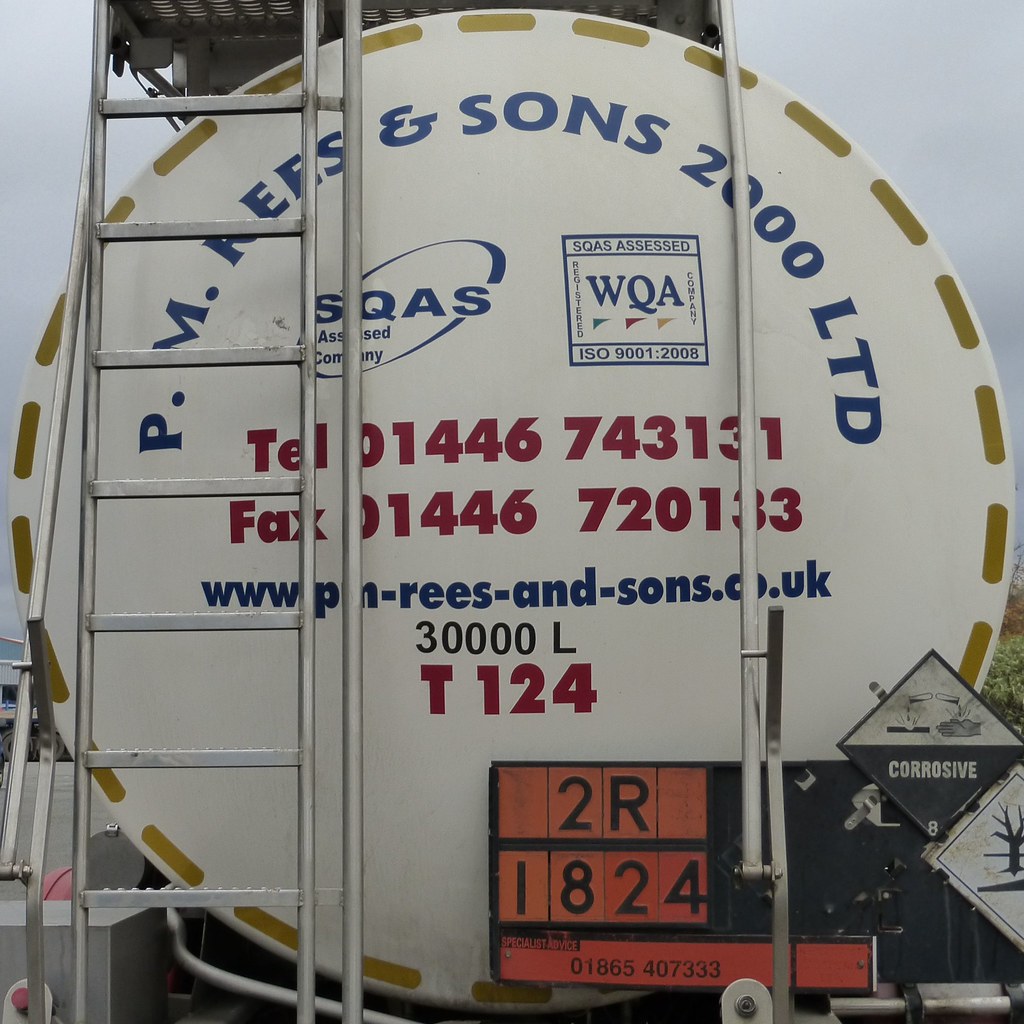This image depicts the side of a large white tank, possibly a tank car, under a gray, cloudy sky. Dominating the center of the tank is a circular sign bordered with dashed gold lines, featuring large blue letters at the top reading "PM REES AND SONS 2000 LTD." Some of the text is partially obscured by horizontal bars but includes additional information such as "SQAS assessed," with a circular logo, and a smaller square indicating "WQA." Below this is bold red text displaying a telephone and fax number, followed by the website address in blue. 

Further down, the tank displays the number "30000 L" with "T124" in bold red beneath it. There are hazard warnings at the bottom right, including corrosive and environmental danger tags. An orange and black sign at the back reads "2R" and "1824," alongside other smaller details. On the left side, there is a vertical metal ladder, positioned probably for maintenance access. This ladder leads up to a black platform on top of the tank, suggesting it's used for filling or emptying the contents.